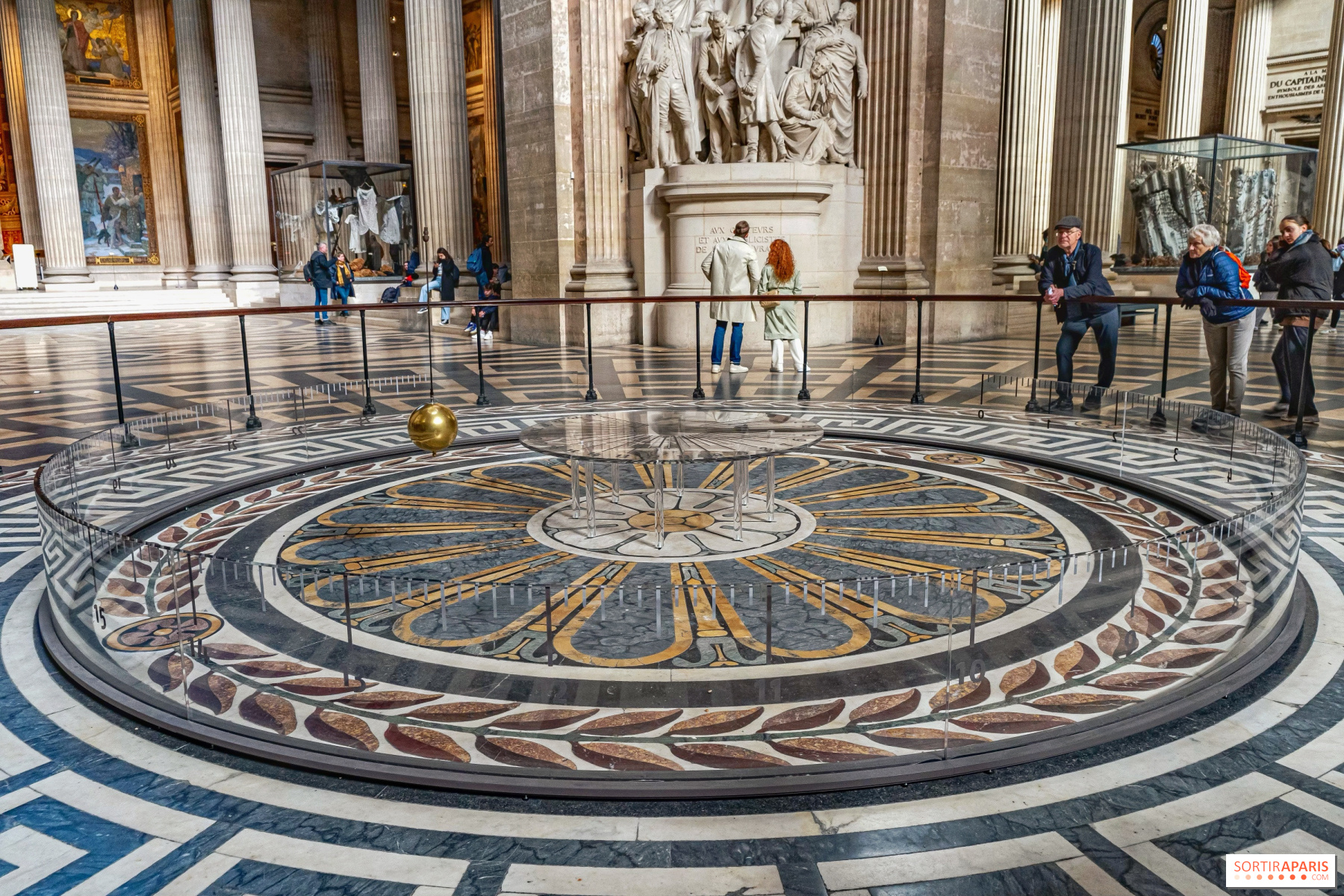The photograph captures the intricate interior of a rotunda within what appears to be a museum or government building. The central focus is a large, brass pendulum encompassed by a circular railing, where three individuals are leaning, observing its steady swing. The floor showcases an elaborate mosaic of bright colors arranged in concentric rings. In the background, a couple stands side by side, their gaze fixed upwards at a grand statue featuring a group of people assembled on a stone structure, possibly representing a historical or artistic tableau. To the left, the space extends into an area where more visitors are seated on steps and ledges, surrounded by additional statues in casings and hanging paintings. The architectural details include tall Doric or Ionic columns adding to the grandeur of the room, which also features delicate blue and gold piping designs. A large glass backing frames part of the scene, further enhancing the sense of depth and complexity in this cultured and historic space.